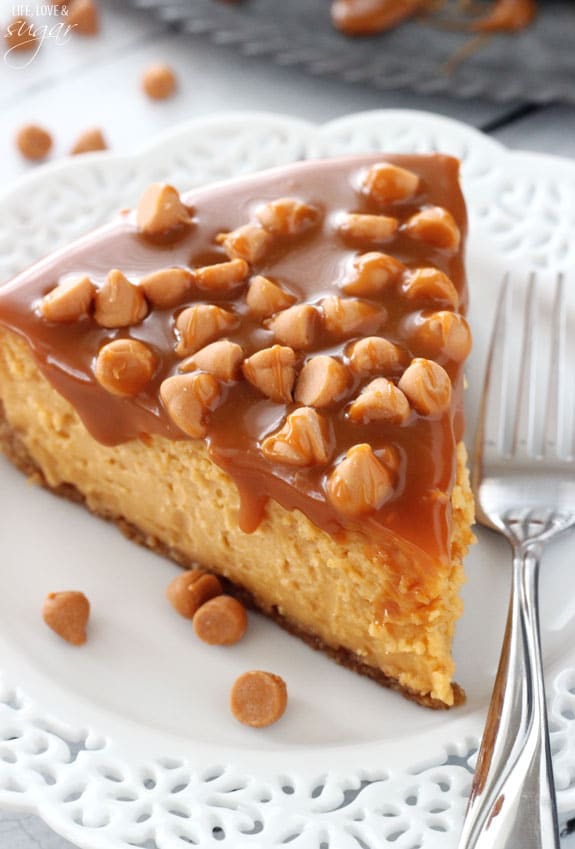The image is a vertical rectangular photograph of a dessert, likely a piece of cake or pie, centered on an ornamental white plate, about 6 inches across. The plate features intricate, lace-like cut-out patterns along its scalloped edges. The dessert is set on a light gray wooden table, which might have a dark gray circular placemat partially visible at the top edge of the image.

The dessert is a wedge-shaped slice, with a yellowish-beige filling that could suggest caramel cheesecake or pumpkin pie. It has a very thin, almost chocolate-looking crust at the bottom. The top of the dessert is drizzled with what appears to be caramel sauce and is sprinkled with tooth-shaped orange frosting nuggets or caramel chocolate chips.

To the right of the plate lies a clean stainless steel fork, its prongs pointing upwards, indicating the dessert has not yet been touched. In the background, there is a blurred gray piece of fabric with something brown on it, adding a subtle layer of depth to the setting. On the top left of the image, the words "Life, Love, and Sugar" are written in white font. Overall, the image captures an inviting and detailed scene of an untouched dessert ready to be enjoyed.